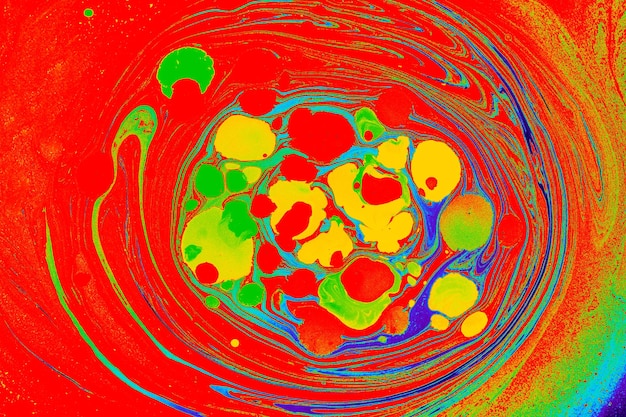The image appears to be an abstract artwork, potentially digital or a painting, characterized by its vibrant and bold use of color, reminiscent of Op Art. The main background is a vivid red, providing a striking contrast to the swirling patterns above it. These swirls predominantly feature green and blue, arranged in semicircular and circular formations. Within these circles, various blotches of color, including yellow, green, and red, create a sense of depth and movement. Some of the blotches overlap and are encircled by wavy blue lines, adding to the dynamic appearance. The right side of the artwork is accentuated with additional swishes of yellow, green, and blue. The entire piece imparts a cheerful and lively impression, with the interplay of colors suggesting a fluid, almost wet surface where blobs of paint appear to float in an oil-like mixture. Overall, the artwork is a vivid and detailed exploration of color and form.